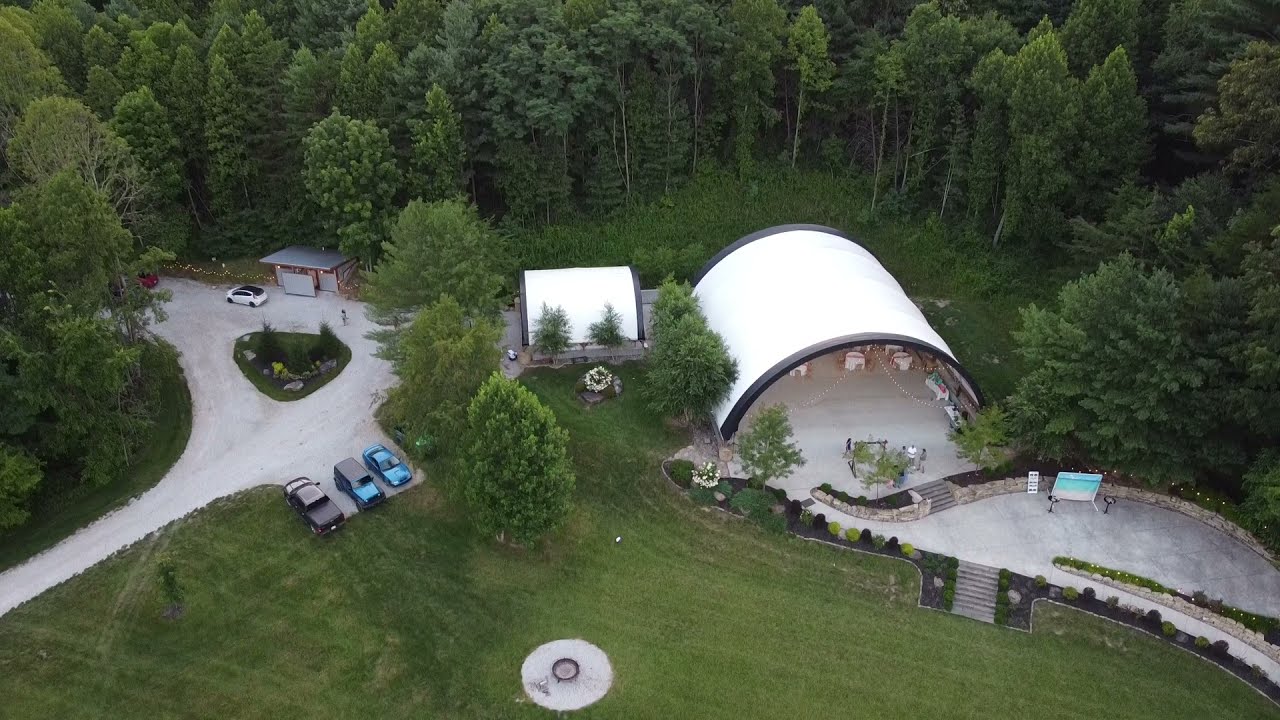The image is an aerial shot of a forested area with a central clearing. Dominating the center of the clearing is a large, dome-shaped white building with black borders, resembling an auditorium or hangar. To the immediate left of this main structure is a smaller white building, possibly a utility facility or bathroom. Surrounding these buildings are tall, lush trees.

A paved Y-shaped pathway leads to the main dome-shaped building, and near its lower right section is a wide concrete pathway and a large square blue screen with a black border. The pathway appears to form an odd shape before reaching the auditorium.

Adjacent to the grass-covered area in front of the main structure is a driveway or road, leading to a small parking lot where three cars are parked. Another small building and a white car are visible in the background. The image showcases clear contrasts: the white structures and concrete pathways against the vibrant green of the surrounding forest and grass.